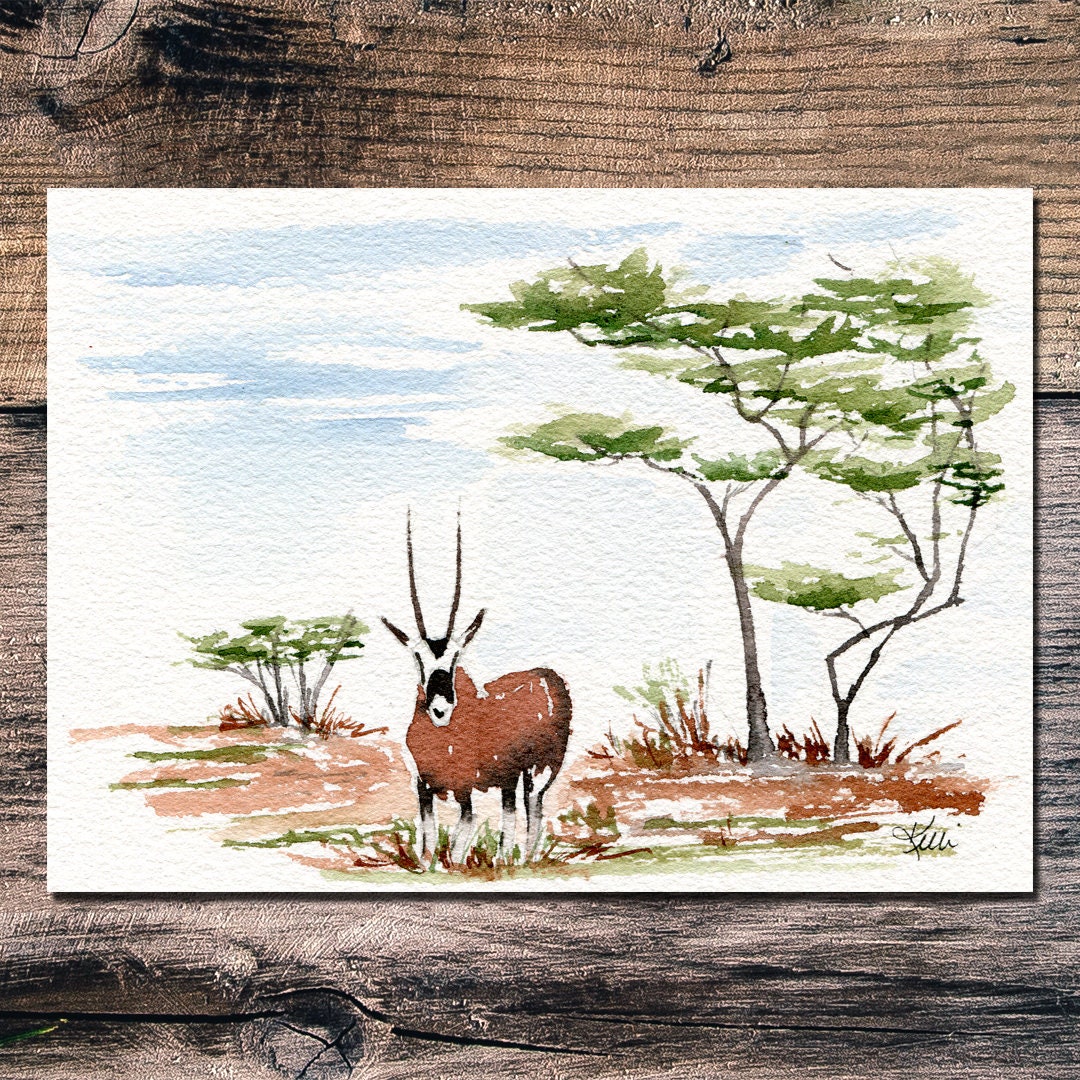This color photograph captures a detailed watercolor painting resting on a backdrop of aged, weathered wood planks, predominantly light brown with some black streaks and a noticeable knot at the bottom. The wood's horizontal grain contributes to the rustic charm. The painting, oriented in a rectangular format, features a white background that uses extensive white space to highlight its subject.

Dominating the foreground is a brown impala, characterized by its distinct white and black face, tall black pointed horns, and upward-facing ears tipped with black. The impala stands on a simple, yet effective representation of grass achieved with strokes of green and brown.

In the background, two trees with light brown branches and green leaves frame the scene, primarily aligned to the right. Above, blue streaks across the top of the painting imply a serene sky, contrasting the stark white background.

In the bottom right corner, the artist’s signature is visible albeit indecipherable, adding a personal touch to this evocative composition.